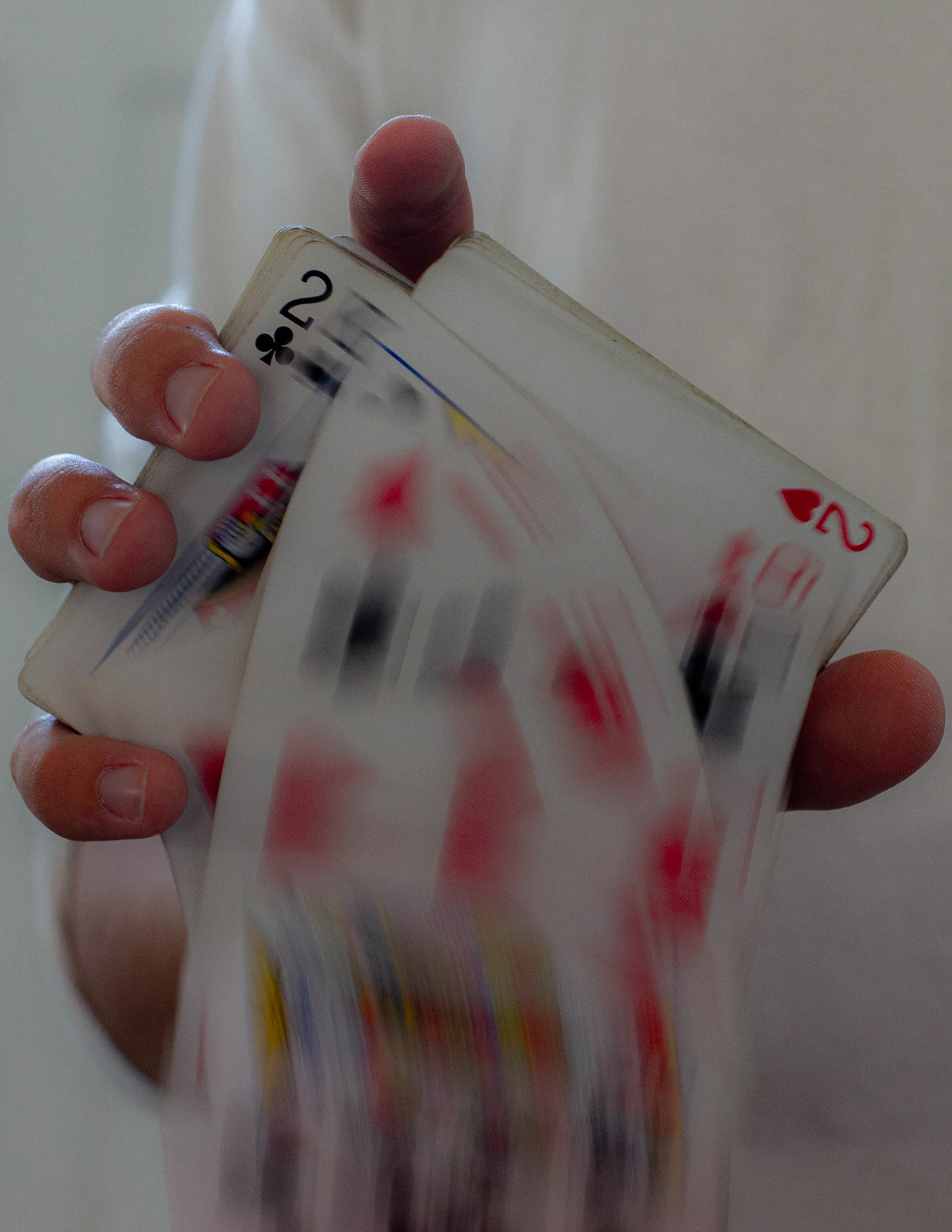Captured in this striking photograph is a dynamic shot of a deck of cards in mid-fall, set against a stark white background. The image, likely taken with a professional camera, features a person wearing a white shirt, with their torso and hand prominently displayed. The hand is positioned towards the camera, gracefully releasing the deck, which cascades downward in a mesmerizing blur. Several cards are discernible amidst the motion, notably a black two of clubs and a red two of hearts. Near the bottom of the image, the blur of colors and shapes hints at other cards, including what appears to be a king or queen, adding to the chaotic beauty of the scene. The overall composition captures the serene yet dynamic moment of the cards' descent, framed perfectly by the simplicity of the person’s white attire and the plain background.